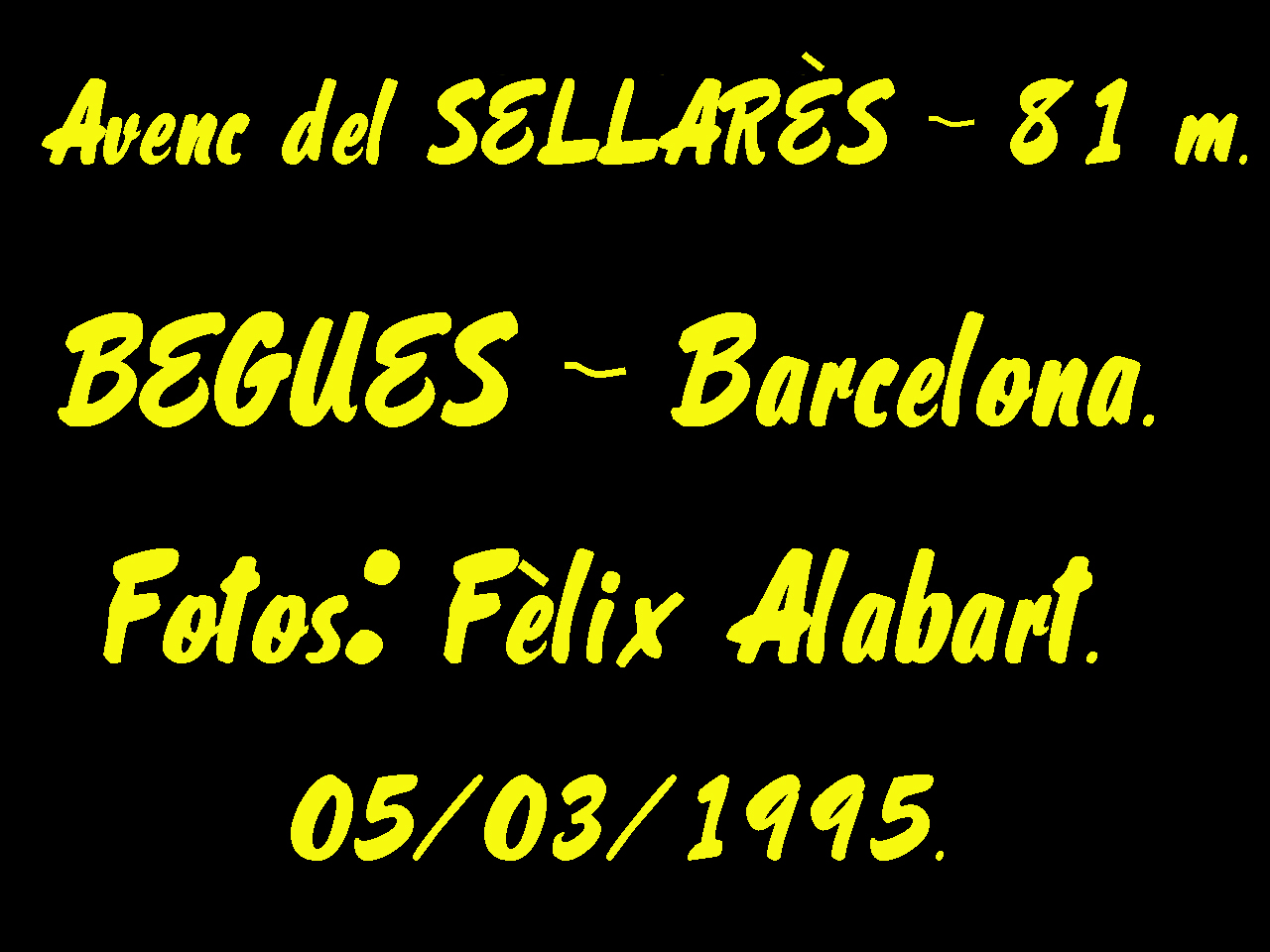The image depicts a landscape-oriented sign with a black background and yellow cursive text. The sign, written in Spanish, reads "Avenc del Celares - 81 meters" at the top. Below this, in uppercase and lowercase letters, it states "Begues - Barcelona." Further down, it mentions "Photos: Felix Alabart" and is dated "05/03/1995." The text appears to be handwritten and stands out vividly against the dark background.